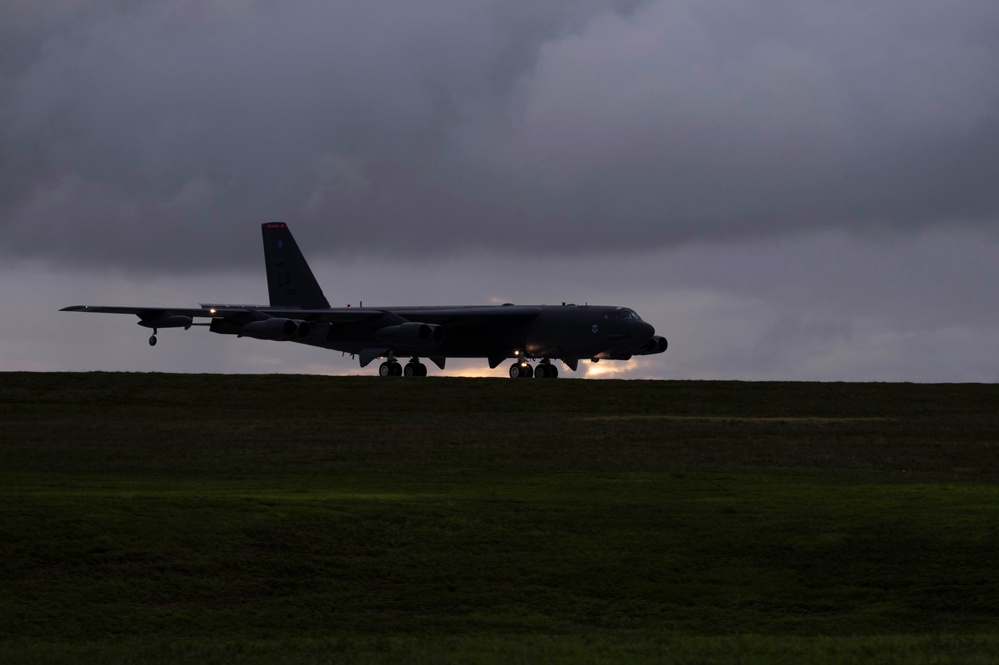This detailed image features a B-52 Stratofortress, a venerable Air Force long-range bomber that has been in service for nearly 70 years. The angle of the shot captures the sleek, black silhouette of the aircraft as it faces the right, possibly preparing for takeoff, just landed, or parked. The sky above is dark and overcast, filled with gray clouds, and the setting sun paints the horizon with a muted glow, suggesting early evening. The runway beneath the plane appears to be minimally visible, blending into the grassy terrain that surrounds it. The hints of light on the aircraft’s tail and wings add depth to the scene, while the overall moody atmosphere hints at a combination of twilight and impending storm. The B-52’s unique, windowless design distinguishes it from commercial airliners, underscoring its specialized military function. There are no other planes in sight, emphasizing the solitary presence of this iconic aircraft.